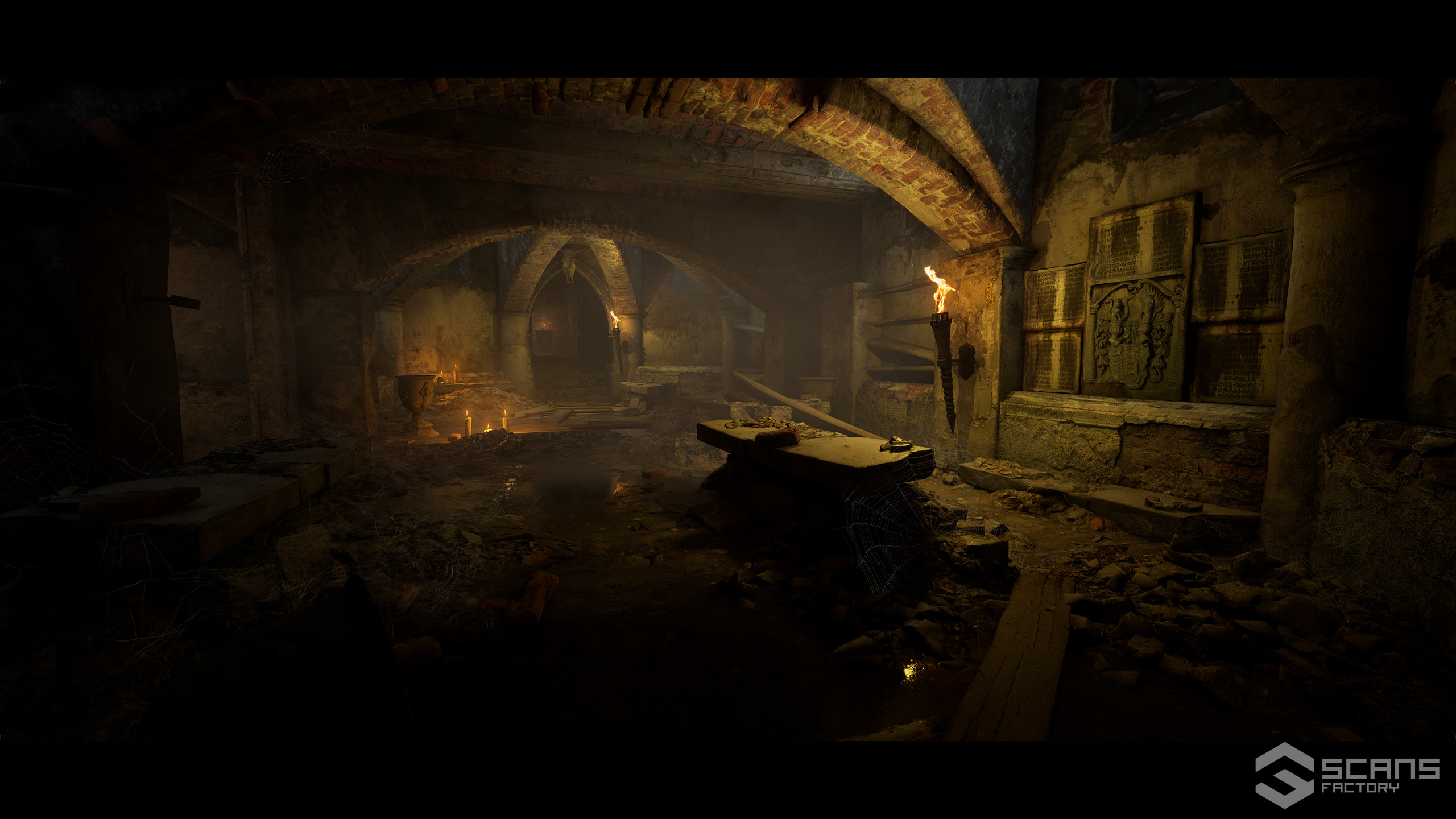The image depicts a dark, dreary interior resembling a dungeon or a secluded section of an old mansion or tunnel. The dominant colors are black, greenish olive, and brown, with an overwhelming sense of decay and destruction. An arched ceiling made of brick rises above the scene, which is heavily cluttered with debris of stones, beams, and crumbled walls. A stone table, appearing almost like a medical table, stands on the right, covered haphazardly with broken stones and chains. The wall on the right, made of cracked greenish stone, looks dilapidated with debris scattered everywhere. Torches are affixed to the walls, casting flickering firelight that barely illuminates the shadowy space. Candles line the floor, contributing to the eerie lighting. In the background, a series of arches are dimly visible, suggesting more of the same desolate atmosphere extends onward. The overall mood is old, creepy, and ominous, further accentuated by the logo "Scans Factory" at the bottom of the image.